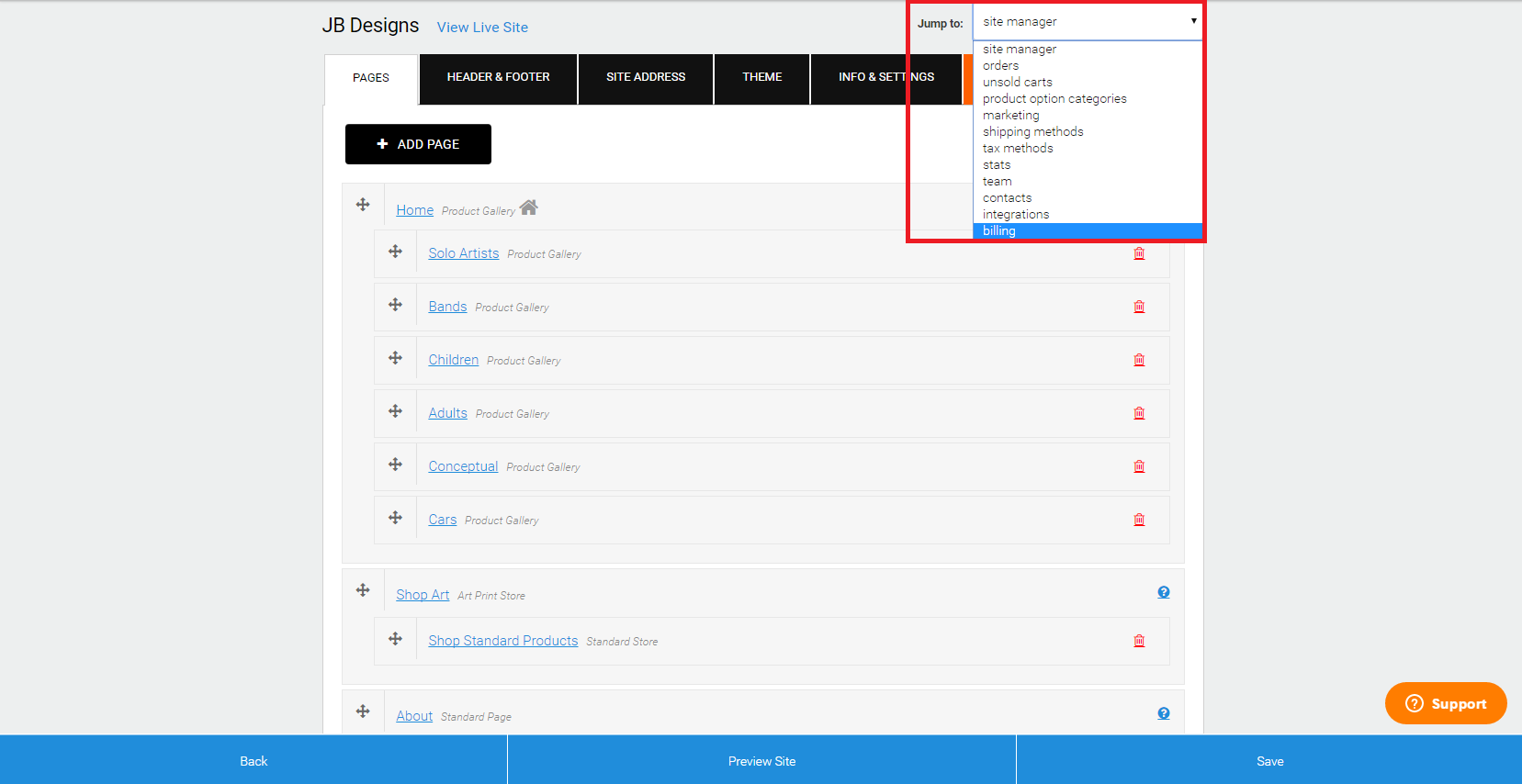A detailed screen capture of the back end of a web design program identified as JB Designs. The interface features a gray background with "JB Designs" displayed prominently at the top left and a hyperlink labeled "View Live Site" to its right. Centered within the gray backdrop is a white section containing a series of five tabs: Pages, Header, Footer, Site Address, Theme, Info, and Settings. Adjacent to these is an orange bar.

Below the tabs, a sidebar on the left side of the screen contains an "Add Page" option with a plus sign, followed by a list of created pages with blue hyperlinks for easy viewing. The listed pages include: Home, Solo Artist Product Gallery, Bands Product Gallery, Children Product Gallery, Adults Product Gallery, Conceptual Product Gallery, Cars Product Gallery, Shop Art, Shop Standard Products, Standard Store, and an "About" link at the bottom.

On the top right, a mini-navigation labeled "Jump To" is situated, featuring a red-outlined white drop-down box displaying various management sections: Site Manager Orders, Unsold Carts, Product Option Categories, Marketing, Shipping Methods, Tax Methods, Stats, Team, Contacts, Integrations, and Billing, with Billing currently selected. To the far right, a column of red trash can icons and blue information dots is visible.

Finally, the bottom right corner houses an orange "Support" button with an adjacent question mark. Across the very bottom of the screen, a blue bar spans the width, showing "Back" on the left, "Preview Site" in the center, and "Save" on the right.